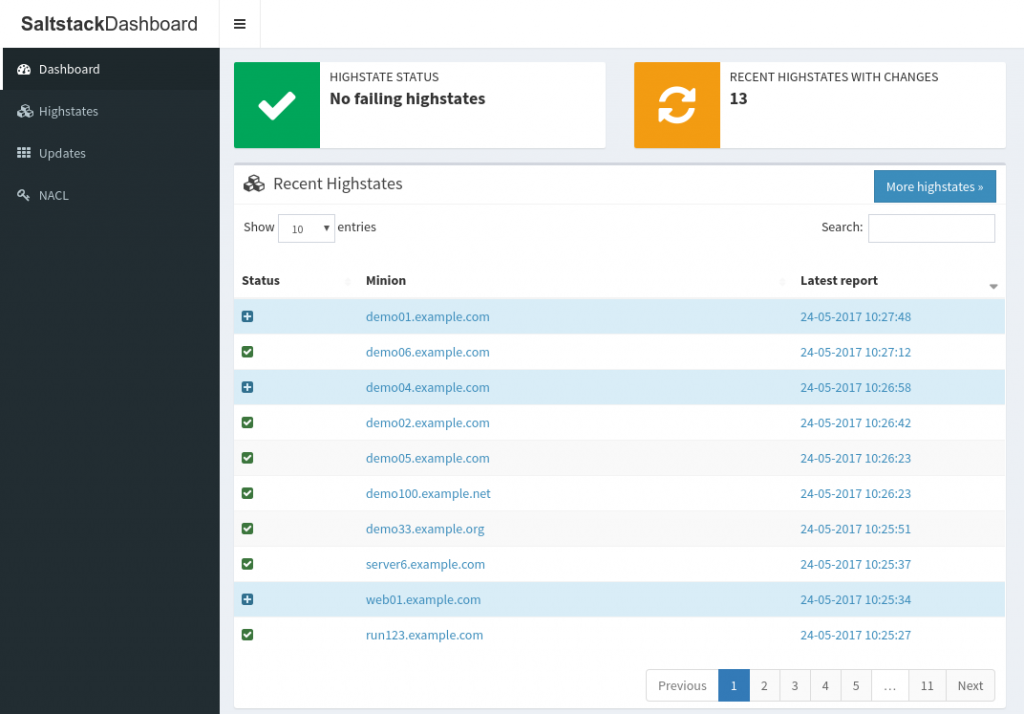The image displays a detailed view of a 'Source Stack Dashboard' interface. The top part of the background is predominantly white, with a black section on the left-hand side, where it is titled "Source Stack Dashboard." Below this title, a gray line runs vertically down, intersected by three horizontal black lines. Another vertical gray line follows, dividing the interface further.

To the left, there is a small black rectangular border containing the text "Dashboard High State Update" in white. Within this rectangle, the word "NACL" is displayed alongside a white key icon.

To the right of this section, there are two rectangles with white backgrounds. The first rectangle features a small green square containing a white check mark. Beside this square, the text reads "High State Status, No Fail in High States." The second rectangle contains a small orange square with two white arrows resembling a refresh symbol. Next to this, the text states "Recent High States with Changes 13."

Below these, spans a larger rectangular box. The left side of this box is mostly white, with the phrase "Recent High States Show 10 Entries" located in the top-left corner. Adjacent to this, on the right side, is a blue rectangle with the white text "More High States." Below that, the word "Search" appears in black. In a white box outlined in gray below "Search," different data columns are presented.

The first column heading reads "Status Minion Latest Report" in black. This column displays status indicators featuring either a blue background with a white plus sign or a green background with a white check mark. The specific pattern shows plus signs for the first, third, and penultimate entries, while the other entries feature the green check marks.